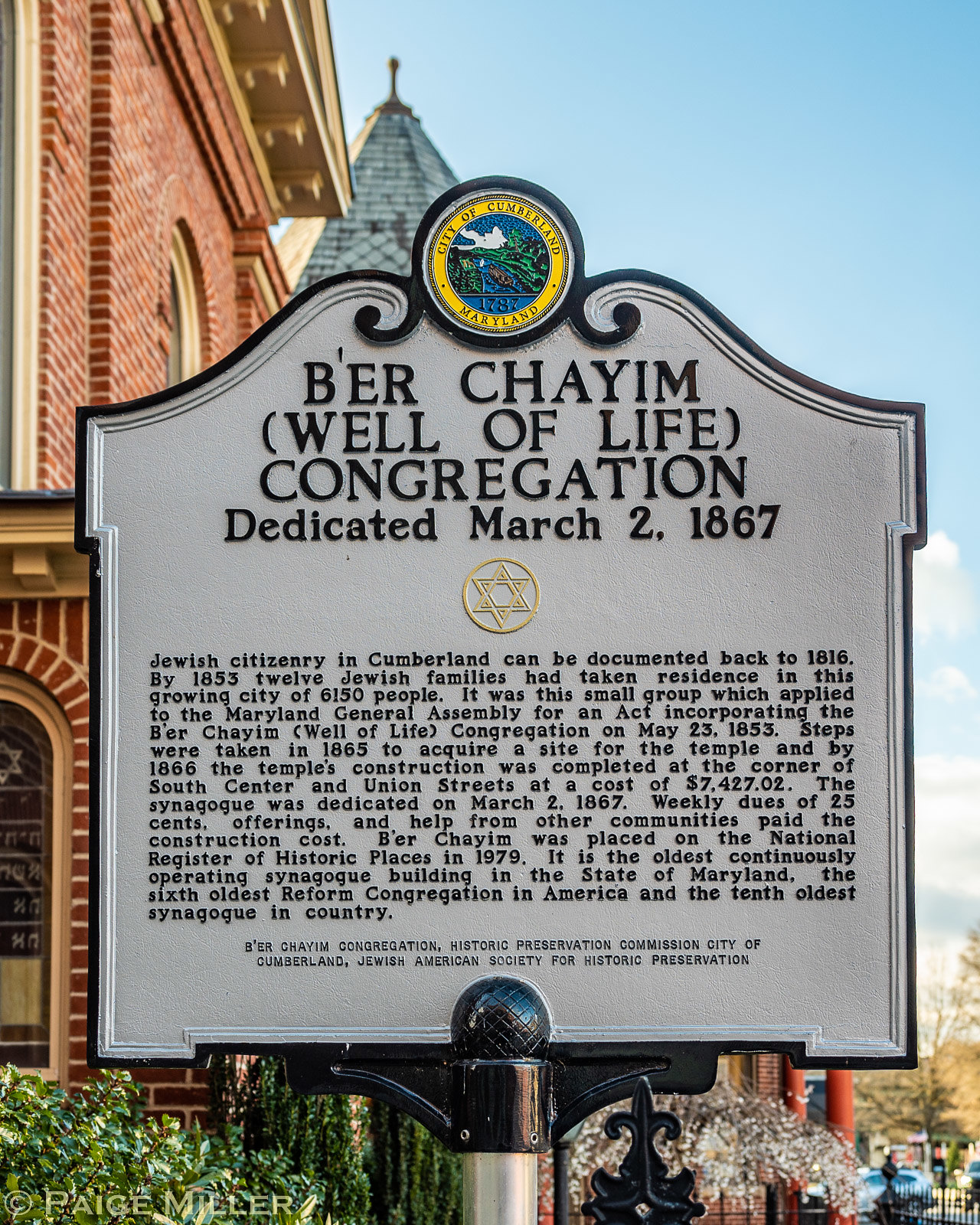This image captures a detailed outdoor scene featuring a historic, ornate black metal sign prominently displayed next to a picturesque red brick building, partially visible to the left. At the top of the sign, a circular insignia reads "City of Cumberland, Maryland" and depicts an artistic rendition of a river. Below this emblem, the sign is titled "B'er Chayim (Well of Life) Congregation, Dedicated March 2, 1867," followed by a Star of David. The main body of the sign contains an informative paragraph detailing the rich history of this Jewish congregation: Jewish citizenry in Cumberland dates back to 1816, with twelve families settled in the city by 1855. These families applied to the Maryland General Assembly for the incorporation of the Well of Life Congregation in 1853. By 1865, efforts began to secure a site for the synagogue which was completed in 1866 at the corner of South Center and Union Streets for $7,427. The synagogue, dedicated on March 2, 1867, was funded through weekly dues of 25 cents, offerings, and community support. It is notable as the oldest continuously operating synagogue in Maryland, the sixth oldest Reformed congregation in the United States, and the country's tenth oldest synagogue. It was listed on the National Register of Historic Places in 1979. The metal sign is mounted on a black fixture attached to a metal pole, grounding it in front of the historic setting. A steeple is visible behind the sign, and glimpses of the sky can be seen to the upper right and far right of the image. The bottom left corner of the sign bears the name "Page Miller."